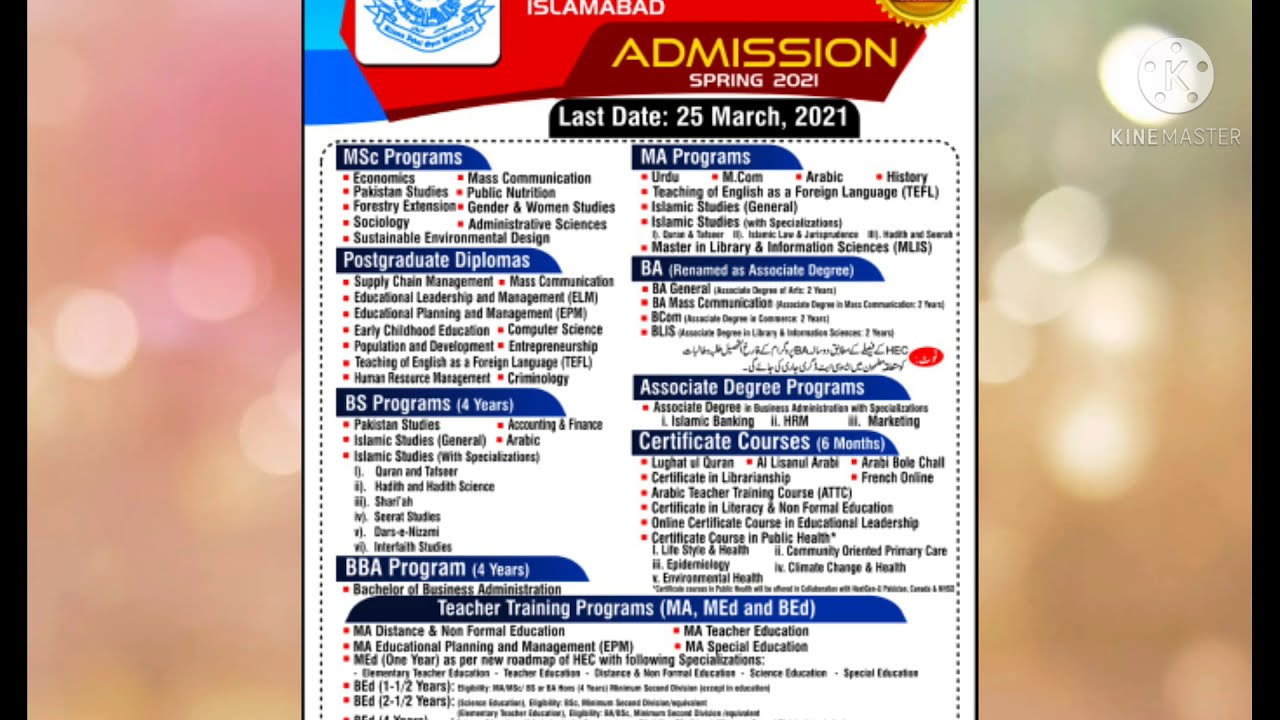This image appears to be a screenshot of an informational graphic designed as a university pamphlet. Dominated by a structured layout, it highlights various academic programs and important deadlines for admissions. At the very top, a red banner with hints of blue houses a partially visible logo along with the text 'Islamabad'. Adjacent to this, in bright yellow and dark red, it states 'Admission Spring 2021'. Below this, in a black text box, the deadline 'Last Date: 25th March 2021' is prominently displayed.

Diving into the details, the graphic categorizes information with blue text boxes. The categories include MSc Programs, listed with courses like Economics, Pakistan Studies, Forestry Extension, Sociology, and more. Next, Postgraduate Diplomas feature options such as Mass Communication and Supply Chain Management. The graphic extends to BS and BBA programs, emphasizing their duration as four years. Further down, Teacher Training Programs are mentioned.

On the right column, programs for MA and BA (renamed as Associate Degree), alongside Associate Degree Programs and Certificate Courses of varying durations, are detailed. The calm, out-of-focus background in beige, peach, and grey, adorned with sparkling objects and bubble-like graphics, suggests a video context, further confirmed by the 'KineMaster' logo in the upper right corner. This cohesive layout indicates a thorough guide for prospective students on academic offerings and application deadlines for Spring 2021 at the university in Islamabad.